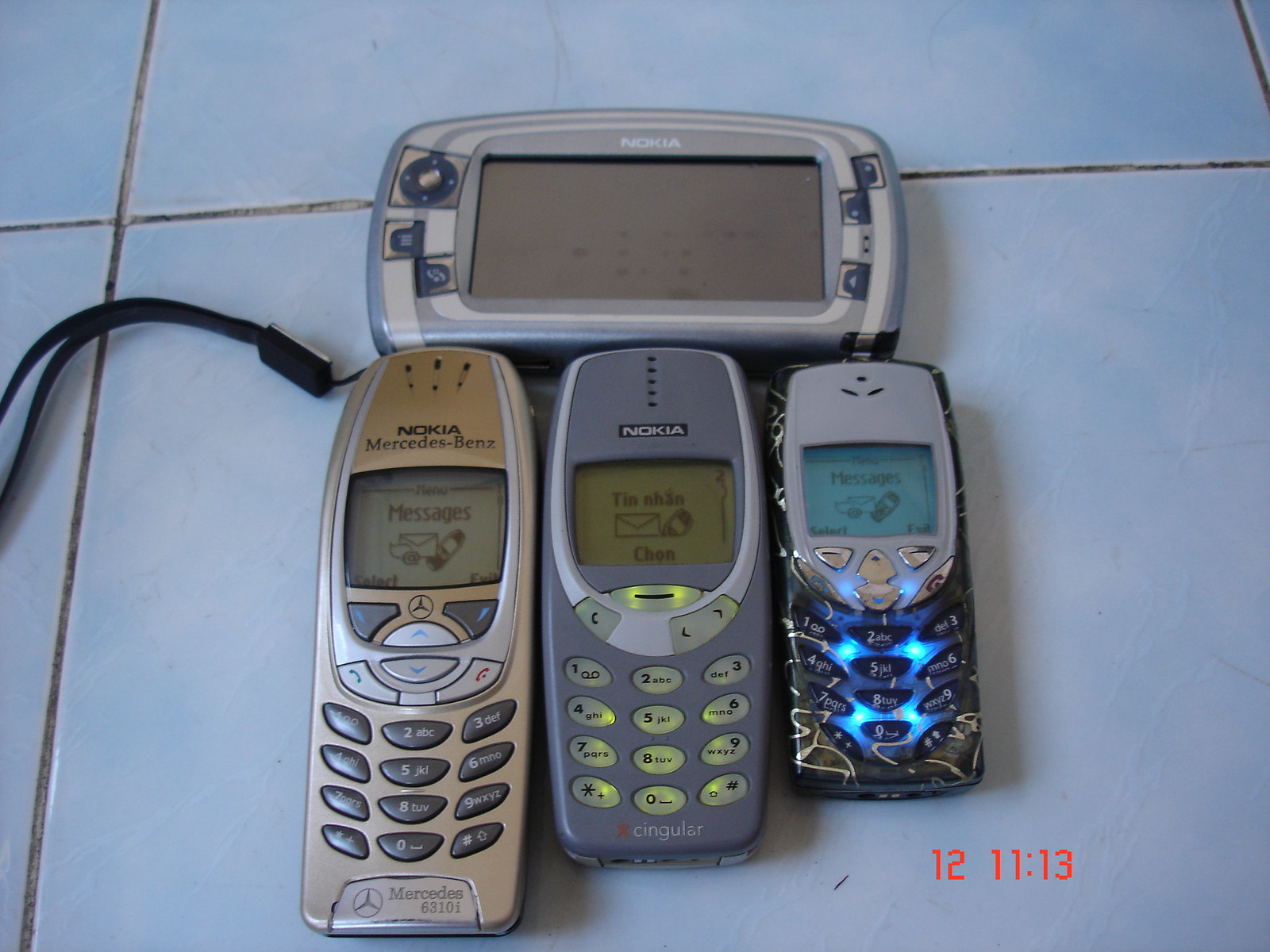In the photograph, a trio of vintage Nokia cell phones are placed on a white tiled background. Starting from the left, the first phone is branded as a Nokia Mercedes-Benz model, suggesting it's an older car phone. It features a distinct grey and dark grey color scheme. The middle phone, slightly larger, sports a grey-blue hue with neon backlighting on its buttons. To the right, the smallest phone has a black casing with blue backlights behind its buttons and a grey screen. Positioned above these phones, there appears to be a handheld gaming system with a black cord attached. Notably, on the bottom right corner of the tile are the numbers "12" and "11.13," possibly marking the date or a specific detail related to the scene.